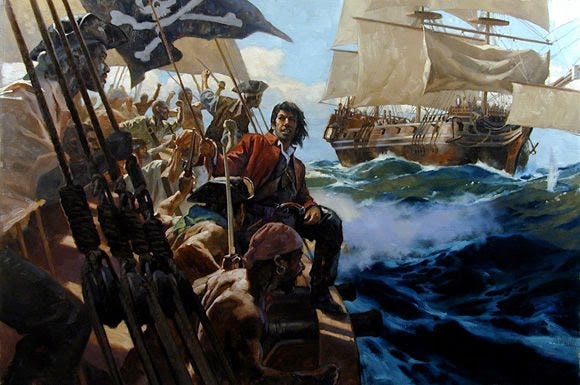This painting vividly depicts an intense maritime scene with two ships contending on a turbulent ocean characterized by dark blue, green, and black waves interspersed with dramatic foamy crests. On the left side of the image, a densely packed pirate ship, flying the iconic black flag with a white skull and crossbones in the upper left corner, is bustling with activity. The pirates, dressed in a mix of long-sleeve shirts ranging in colors from white to rust orange to brown, are animatedly clustering towards the right, seemingly fixated on the approaching vessel. At the forefront, a striking figure in a red coat, white shirt, and black boots stands out prominently; his left foot is braced on the edge of the ship with his elbow resting on his knee, embodying an air of readiness and defiance. Below him, a motley crew of sailors, some in rags and varying headgear, raise their fists in fervor. To the right, in the upper corner of the painting, a larger and less populated brown ship with expansive white sails looms. This ship, outfitted with numerous cannon ports, appears to be the focus of the pirates' attention. Adding to the tension of the scene, a plume of smoke rises from the middle of the composition, hinting at the imminent clash between these two vessels.